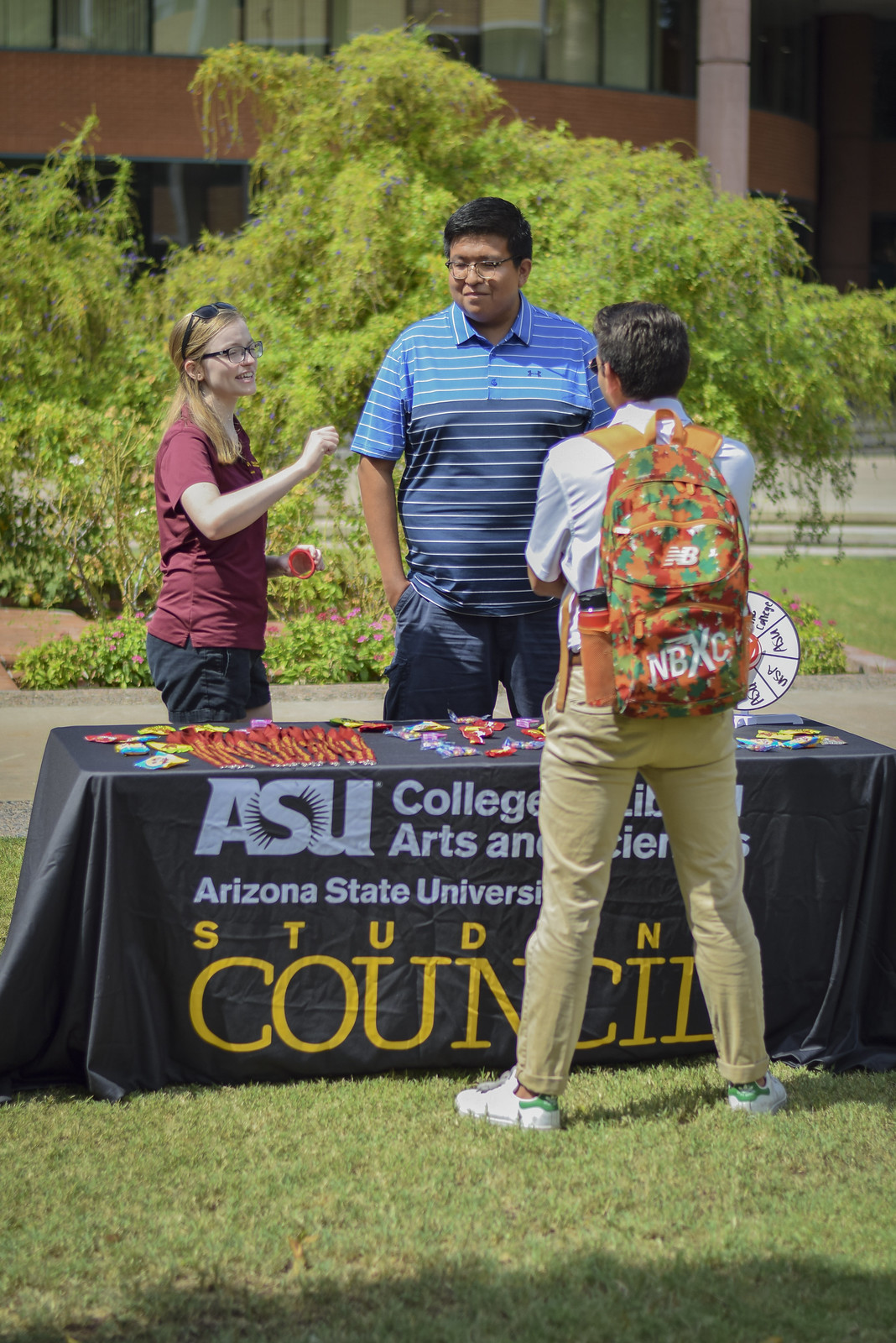In this outdoor midday image, set against a grassy lawn at Arizona State University, a small table with a black tablecloth emblazoned with "ASU College of Liberal Arts and Sciences, Arizona State University Student Council" stands at the center. Surrounding the table, three individuals are engaged in conversation. Two of them, a young woman and a man, face a third individual seeking information. The young woman, positioned to the left, sports long dirty blonde hair, glasses, a red t-shirt, and black shorts. Beside her, a larger man in a light blue and navy blue collared shirt stands. The inquiry is being made by a man sporting khaki pants, a white shirt, an orange backpack, and white and green Stan Smith sneakers. The scene is complemented by a backdrop of lush green grass, a nearby bush, and a distant building, with various colors like green, brown, black, gray, yellow, orange, purple, and tan vividly noticeable. Small knickknacks and a spin wheel are also visible on the table, suggesting a typical college orientation event.